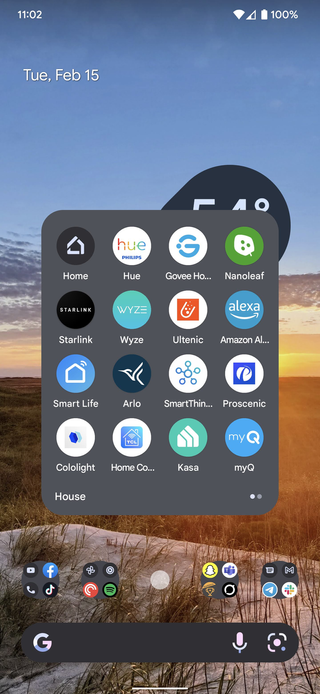The home screen of an Android phone is meticulously organized with a unique layout. At the bottom, the Google Assistant search bar provides easy access for typing on the large screen. Four groups of icons dominate the bottom row, each containing four app icons, including popular apps like Spotify, Snapchat, Gmail, Pocket Cast, TikTok, and Facebook. In the middle of the screen, there's a larger folder with at least 16 app icons, featuring various smart home applications such as Wise, MyQ, Hue, Starlink, and Amazon Alexa. This folder, labeled "House" on the bottom left, aptly organizes all home-related apps, streamlining access to smart home controls. Swiping right reveals even more categorized apps, reflecting a highly organized and efficient home screen setup.